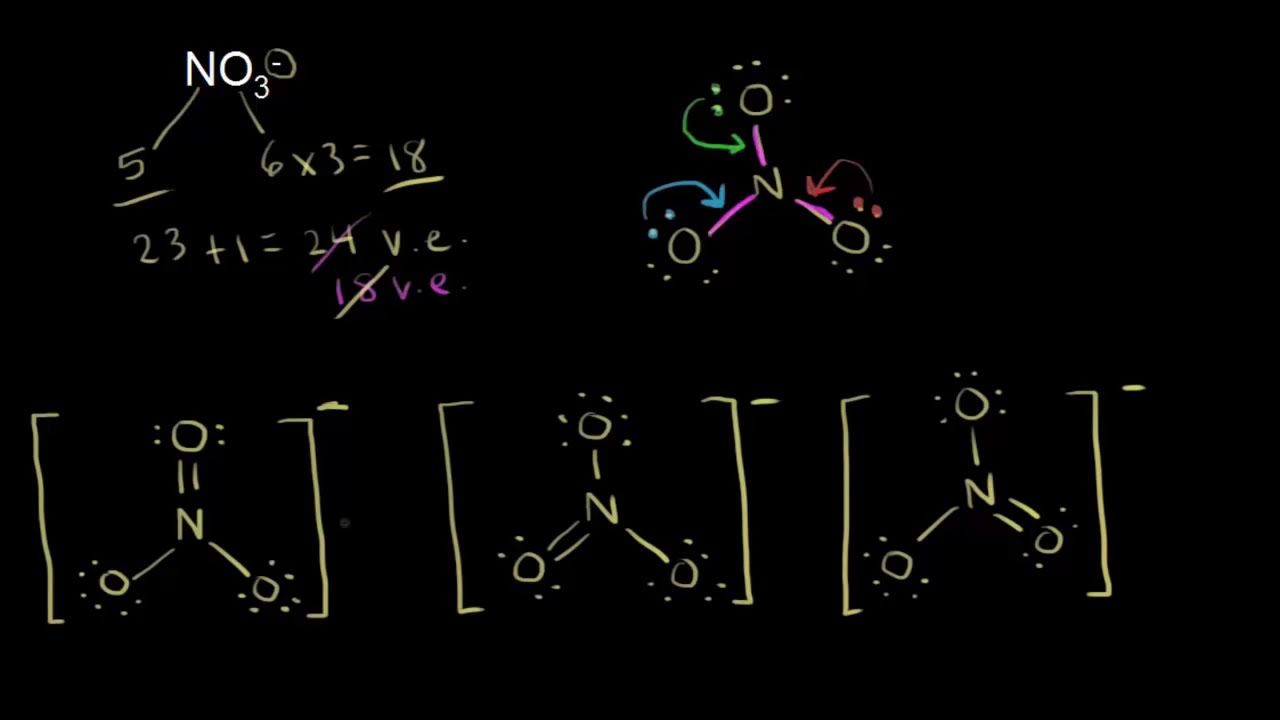The image depicts a dark gray or black background resembling a classroom chalkboard, covered in multi-colored chalk markings depicting a complex chemistry equation or lesson. In the top left corner, "NO3" is prominently written in white. Below it, there are several mathematical equations: "5" with an arrow pointing to "6 times 3 equals 18," "23 plus 1 equals 24,” and “24” crossed out in purple, alongside "18VE" also in purple font.

To the right, three lines emanate from an "N", each line capped with an "O" and surrounded by differently colored dots (green, blue, and red) and arrows of matching colors. Below this arrangement, three "N" figures are depicted, each with varying numbers of lines above and below them, topped with circles and dots, suggesting molecular structures or bonding patterns.

The overall scene looks like a chemistry lesson with elements and equations scribbled in yellow, red, blue, pink, green, and purple chalk, contributing to an advanced scientific explanation or classroom instruction.